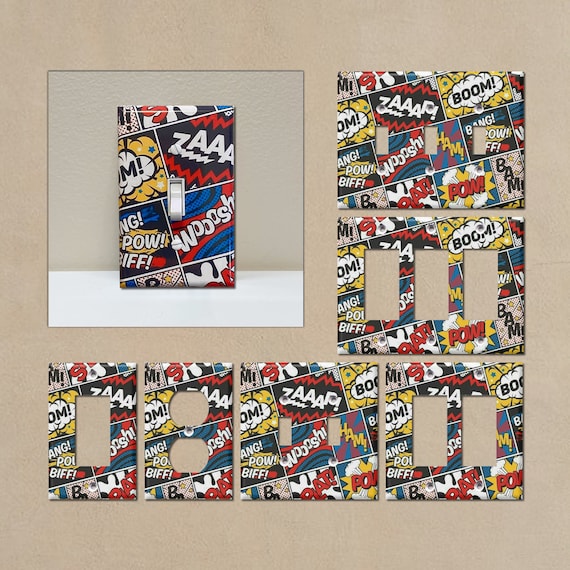The image features a beige square background with a smaller square positioned in the top left corner, which contains various designs of light switch plates and outlet plates. These plates are rectangular and come in different configurations, including ones with two and three switch openings, as well as button switch and outlet plate designs. The plates are adorned with vibrant, comic book-style graphics that include bold text such as "ZAP," "BOOM," "WHOOSH," "BAM," "POW," "PAL," "RIF," "BANG," and "SLAM." The color palette predominantly uses primary colors—red, blue, yellow, along with black and white. White lines separate the different captions, emphasizing the dynamic, cartoonish aesthetic. The overall design evokes the playful and energetic feel of a comic strip, creating a lively and engaging visual experience.